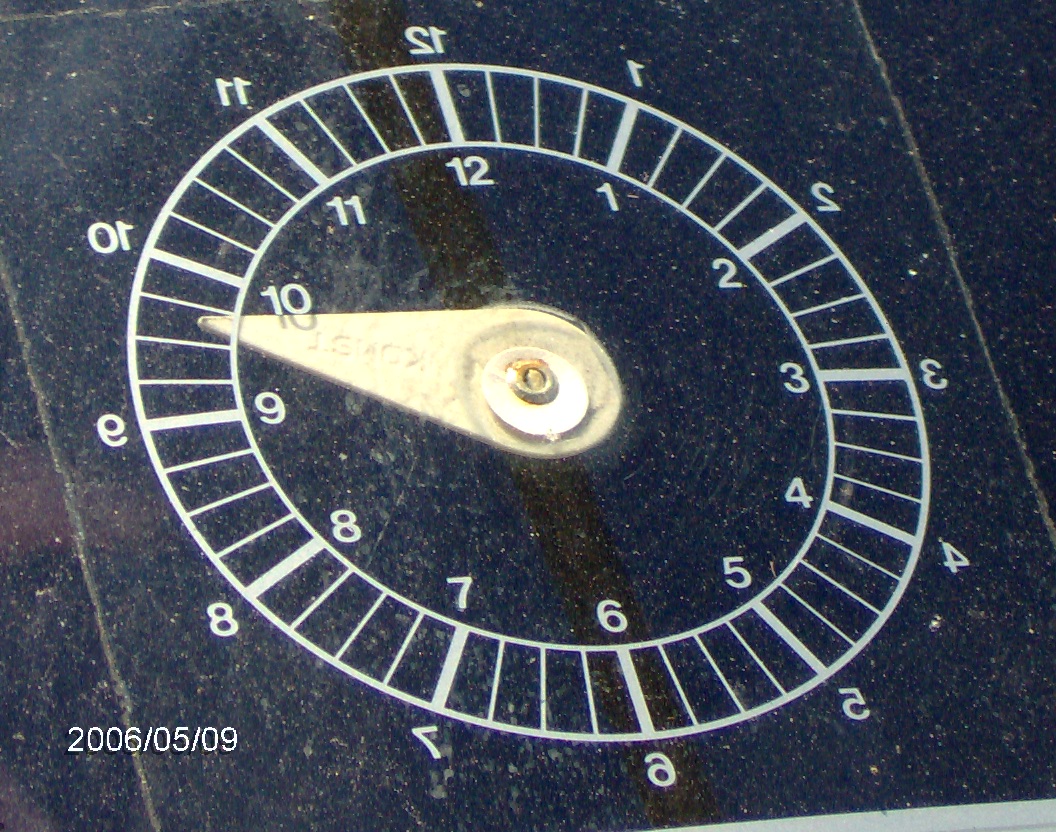This photograph features a peculiar clock positioned on the ground, creating an unusual visual effect. The clock face includes two sets of numbers: the outer set, which are mirrored and appear reversed (for instance, '21' instead of '12'), and the inner set, which follows the conventional arrangement from 1 to 12. Notably, there is no separate hour or minute hand; instead, a single substantial beige hand spans the clock face, pointing just before the 10 mark. This thick hand is anchored by a golden bolt in its center, giving the impression that the entire clock might be embedded in a black icy surface. Adding to the surreal quality of the image, the clock almost seems to be painted or projected onto the ground rather than being a tangible, freestanding object. The bottom left corner of the photograph displays a date, "2006 05 09."